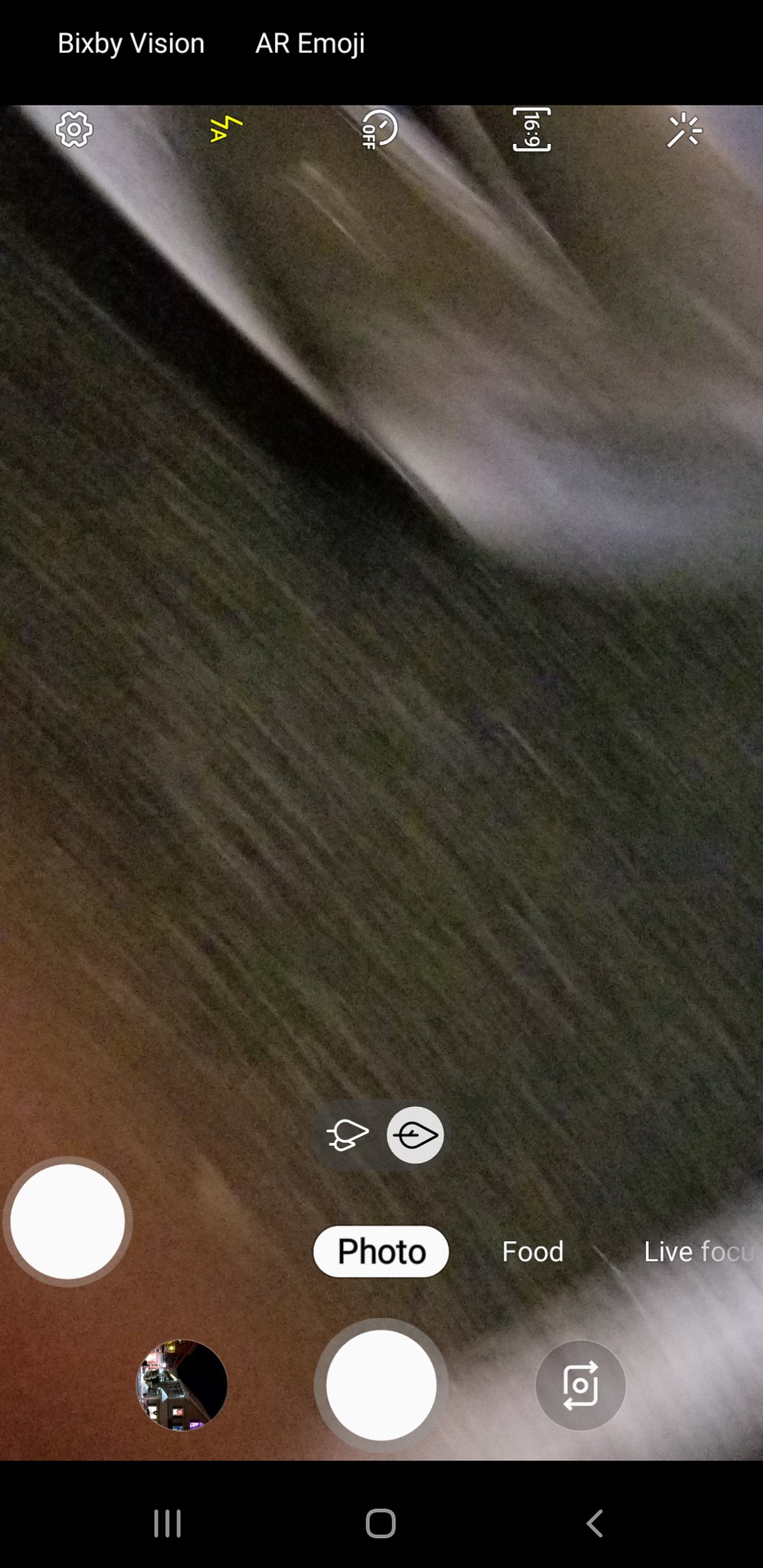This color photograph, evidently taken with a smartphone camera, presents a highly blurred and indistinct scene. The image features a dark, almost black area at the center, flanked by gray sections near the top and lower right-hand corner. The interface overlays for the camera are visible, indicating the use of photographic functions. At the top left of the screen, "Bixby Vision" and "AR Emoji" options are displayed. Toward the bottom, various camera function icons are present, including those for taking a photo, a specialized food photo setting, and a live focus mode. The image is in portrait orientation, revealing no discernible people or animals within this unclear capture.